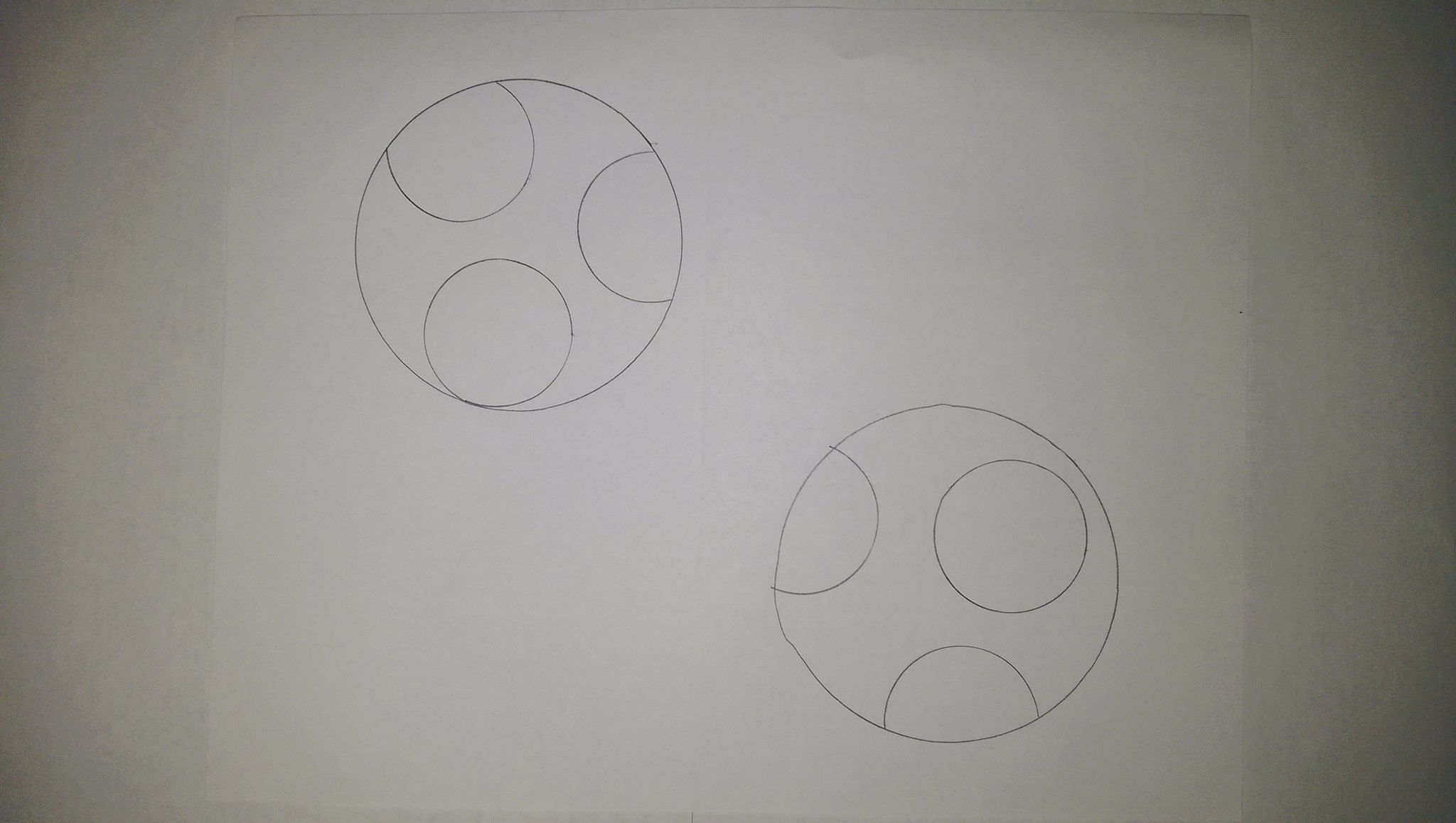This image appears to be meticulously hand-drawn on white paper, utilizing a protractor for precision in most areas. The illustration features two large circles, one positioned at the top left and the other at the bottom right of the page. The top left circle is notably symmetrical and impeccably round, showcasing careful attention to detail. In contrast, the bottom right circle, while still largely symmetrical, deviates slightly from perfect roundness, exhibiting a small jutting area that disrupts its otherwise smooth perimeter.

Within each of these two large circles are three additional smaller circles, each seemingly drawn with the same precision tool. In both the top left and bottom right circles, one of the smaller circles is a complete, perfect circle. The other two smaller circles in each set are partially truncated, as their boundaries intersect with the outer edge of the main circles. This truncation gives them the appearance of half or three-fourths circles.

The slight imperfection in the bottom right circle creates an uneven distribution of space, making the enclosed smaller circles appear to have more breathing room compared to those in the top left circle. This difference in space adds a subtle asymmetry to the overall composition, making the top left circle appear more harmonious and balanced in comparison.